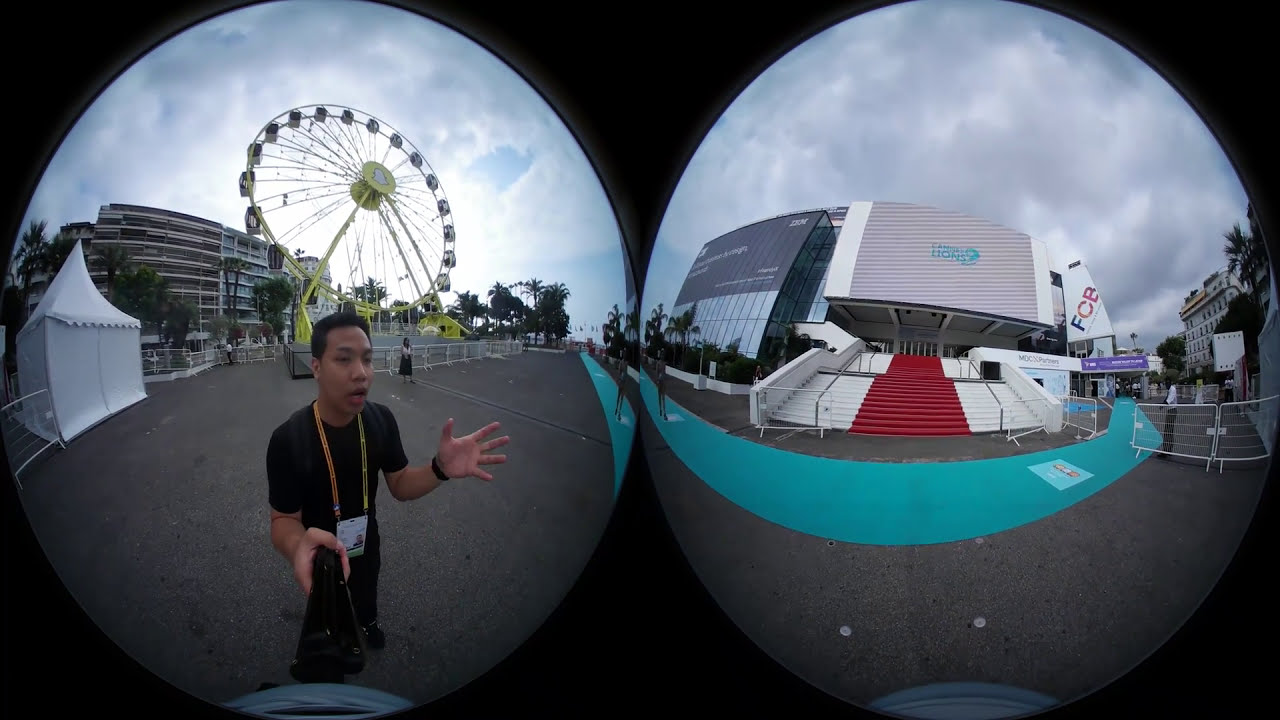The image captures a lively outdoor scene at an amusement park or fair, split into two fisheye lens perspectives. On the left side, a man with black hair, wearing a black t-shirt and a lanyard with a badge, is seen using what appears to be a selfie stick or a GoPro, looking slightly shocked while pointing outwards. Behind him stands a large yellow ferris wheel enclosed by fencing, and a white tent structure is visible beside it. A few palm trees and another building are also discernible in the background under a cloudy gray sky.

The right side of the image offers a view of what the man is looking at: a prominent white building adorned with red and white stairs leading up to its entrance. To the right of this structure, a small gate blocks off access, with a man visible behind the gate. The building features some unreadable text, though a noticeable flag or sign on the right side contains the letters "FCB." Further to the left, there's another mostly glass-front building with dark gray and clear panels. A blue path stretches in front of these buildings, set against a green and blacktop cemented walkway. Various elements, including texting and fencing, appear to be sectioning off areas around the ferris wheel and buildings, implicating a structured layout amid the fairground's bustling backdrop.